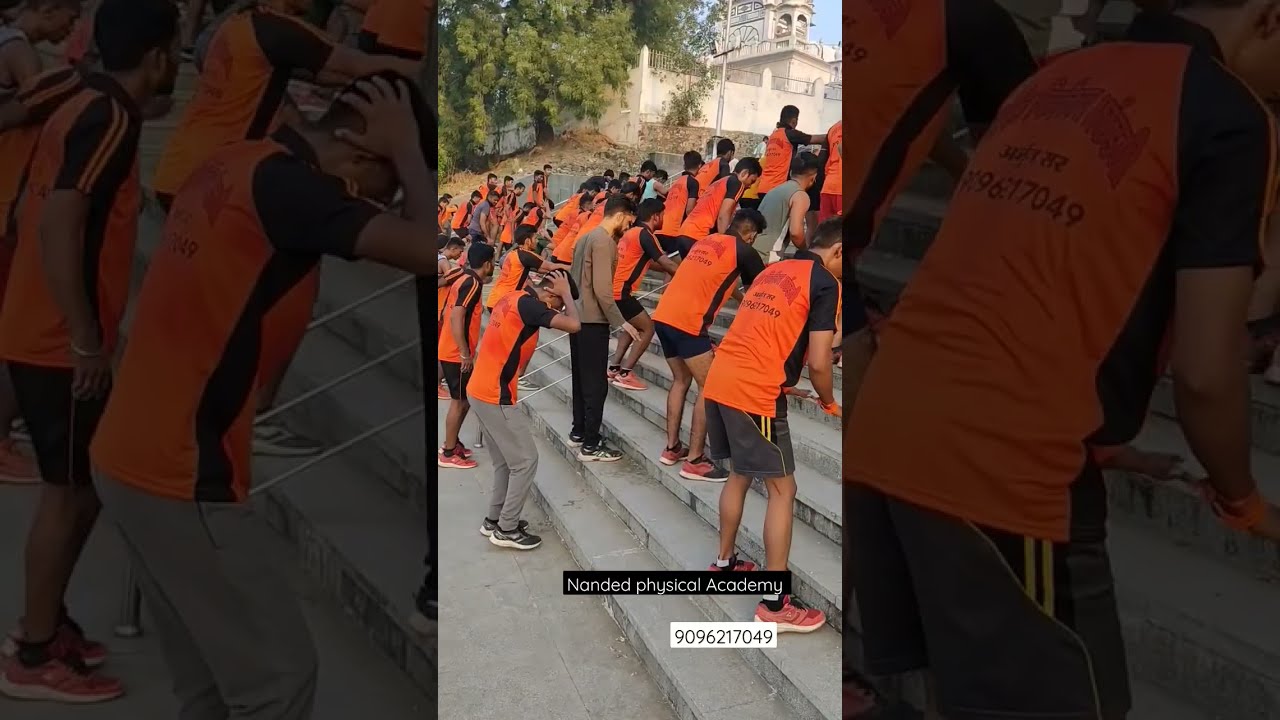In this horizontal rectangular image, the central focus is a group of men, primarily wearing orange and black tops paired with either black or grey athletic shorts and sneakers, some variations include a few in brown athletic pants and long black pants. They are positioned on ascending stone steps, their bodies slightly bent forward as if engaged in a synchronized exercise or ritual. The scene is flanked on either side by faded, close-up sections of the same image with darker backgrounds, highlighting the men in half-lighting. A mixture of greenery from tree canopies is visible on the left side, while a tall stone building contrasts on the right under a bright blue sky. At the bottom of the image, there's a black box with white text reading "Nanded Physical Academy," accompanied by a white box with black text displaying the number "909-621-7049." The composition and layout suggest an organized physical activity on the steps with natural and architectural elements in the background.